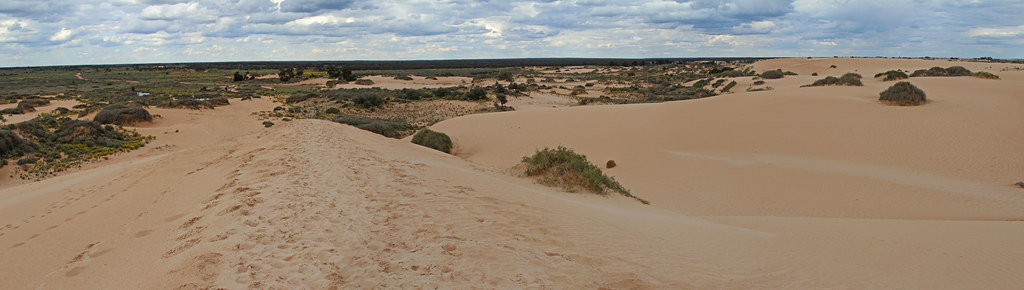The photo showcases a vast desert expanse with no buildings in sight, characterized by a primarily sand-covered landscape with hues ranging from brown to almost orange. The foreground prominently features the sandy terrain with sets of footprints meandering from the left side and trailing off into the distance. As the eye moves further into the background, the scene transitions to patches of green, including bushes, shrubs, and grassy areas, indicating a slight increase in vegetation. This subtle greenery provides a contrast to the otherwise barren foreground. Above the landscape, the sky is filled with clusters of blue clouds with some light and patches of clear sky peeking through, adding depth and ambiance to the daytime desert scene. The overall image captures the diversity and beauty of a desert climate, reminiscent of the Southwest United States, blending arid expanses with hints of flourishing vegetation under a partly cloudy sky.